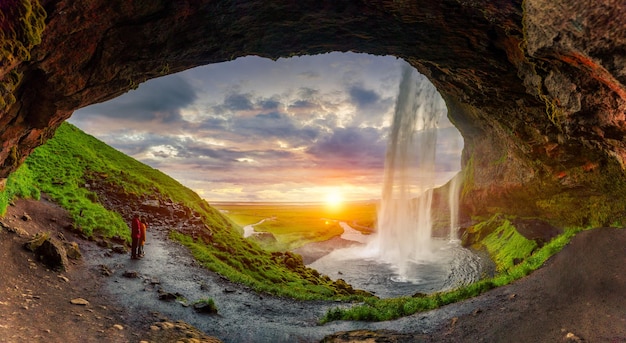The image captures a stunning landscape from the perspective of someone positioned behind a large, rocky grotto, through which a majestic waterfall cascades down into a serene lake before flowing out into a river. The scene is bathed in the warm hues of a breathtaking sunset, casting purplish and bluish tones across the skies and highlighting the lush greenery of the valley. The rocky structure of the grotto, tinted with red, creates a captivating frame for the waterfall. In the bottom left corner, a couple stands together, one in an orange coat and the other in a red coat, mesmerized by the tranquil panorama. Despite some areas being rocky and dark, patches of bright grass punctuate the landscape, contributing to the vibrant and lively atmosphere. The overall image evokes a profound sense of calmness and natural beauty.